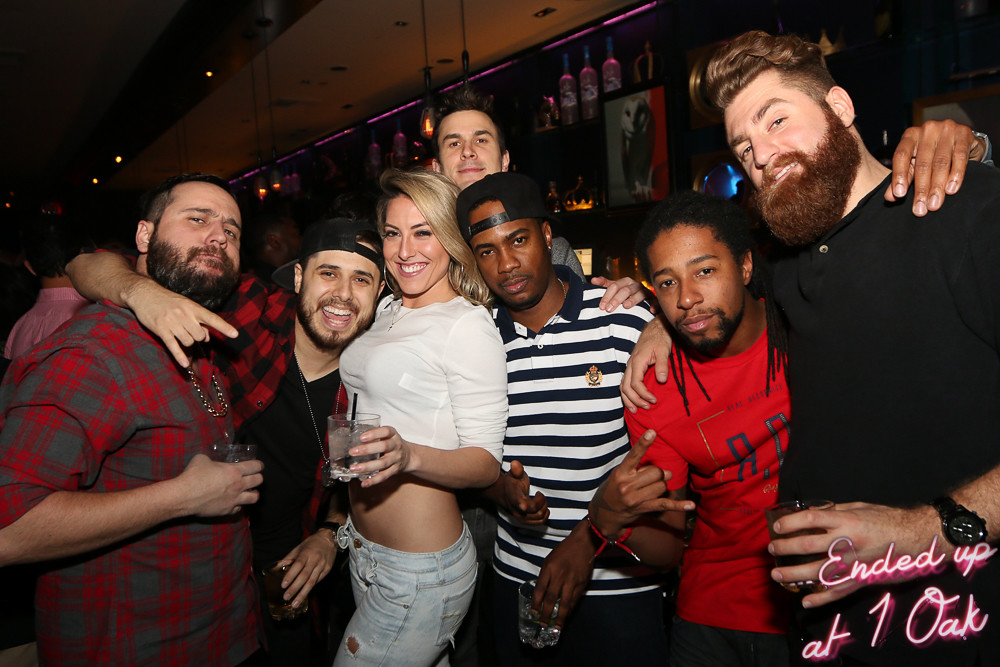In this lively and dynamic group shot taken at the dimly lit bar "One Oak," seven people are having an exhilarating night out. Neon pink text in cursive at the bottom right corner reads "ended up at One Oak," enhancing the energetic atmosphere with neon pink lights against the dark ceiling and walls adorned with shelves of various liquor bottles. In the center, a striking blonde woman in a tight, cropped white halter top and light jeans stands out, holding a drink. Flanking her are six men, all bearded except one. To her immediate left, a white man with a gray and red plaid shirt and a full beard holds a drink in his right hand. To her immediate right, a black man sporting a backward black baseball cap and a black-and-white striped polo shirt stands out. Another white guy with a beard and a black backward baseball cap, wearing a black shirt under a red plaid shirt, is also seen near her, holding a drink in his left hand. Behind them, a man peeks his head above with a smile, adding to the packed crowd. Further to the right, a black man with long dreads, a red t-shirt, and a black beard flashes a devil horns sign with his right hand. His arm is around another man with a big red beard in a black long-sleeve t-shirt, who holds a drink in his left hand. The joyous vibe and varied expressions on their faces reflect a night well celebrated.